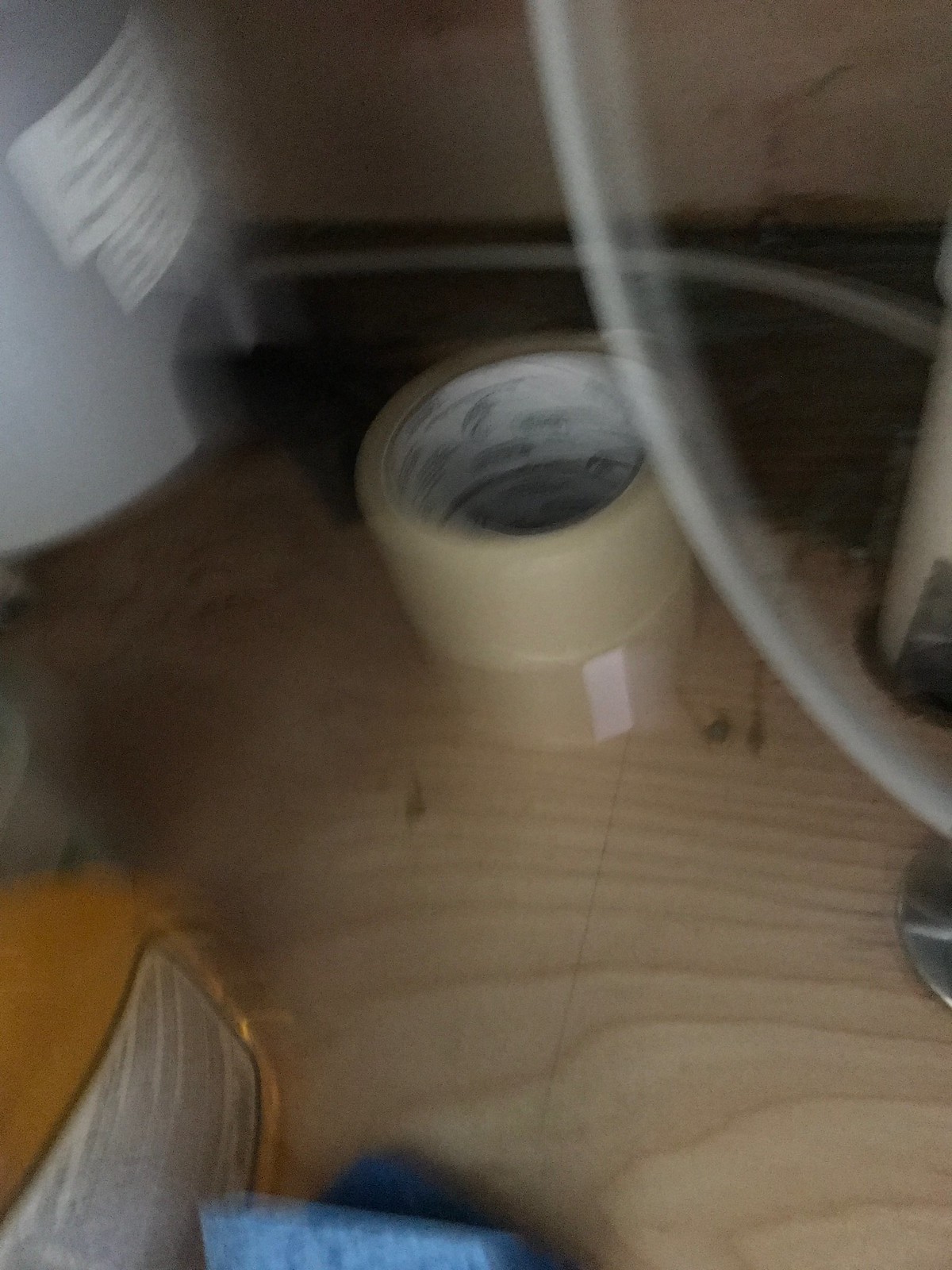The photograph depicts a utilitarian workspace, likely situated under a sink in a dimly lit area. Resting on an unfinished wooden surface are two rolls of tan packing tape, each with a white cardboard core, stacked one on top of the other. In the foreground, the edge of a blue sponge is subtly visible. The background features an obscure appliance with various tubes extending from it and a white-labeled cylinder that remains unreadable. An orange item, possibly part of the sponge or a separate object, is also faintly discernible. A power cord winds through the scene, descending from the top right and wrapping around an unidentified structure before connecting with the cylinder on the left. The image, although blurry, captures an essence of practicality and disarray.